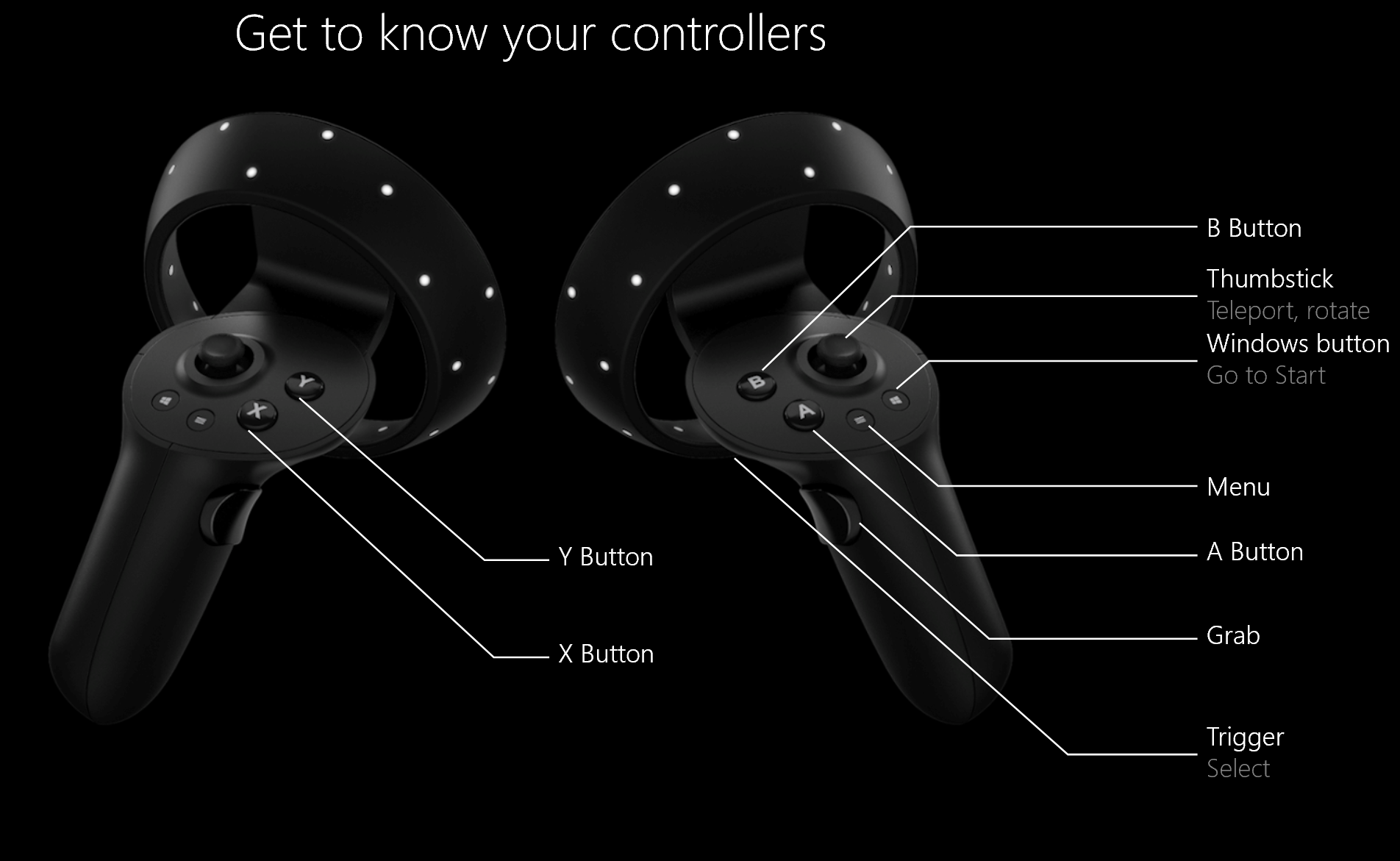The image features two black VR controllers with a black background. At the top of the image, white text reads, "Get to know your controllers." Each controller has multiple lines pointing to its various buttons and functions. To the right controller, labels identify the B button, thumbstick (used for teleport and rotate functions), Windows button (go to start), menu button, A button, grab button, and trigger (used to select). The left controller identifies the Y and X buttons, situated accordingly. Both controllers are dark in color, with white dots along the top, possibly designed to help the features stand out. Every button and command is clearly annotated in white lettering, providing comprehensive detail about the controllers' functions.